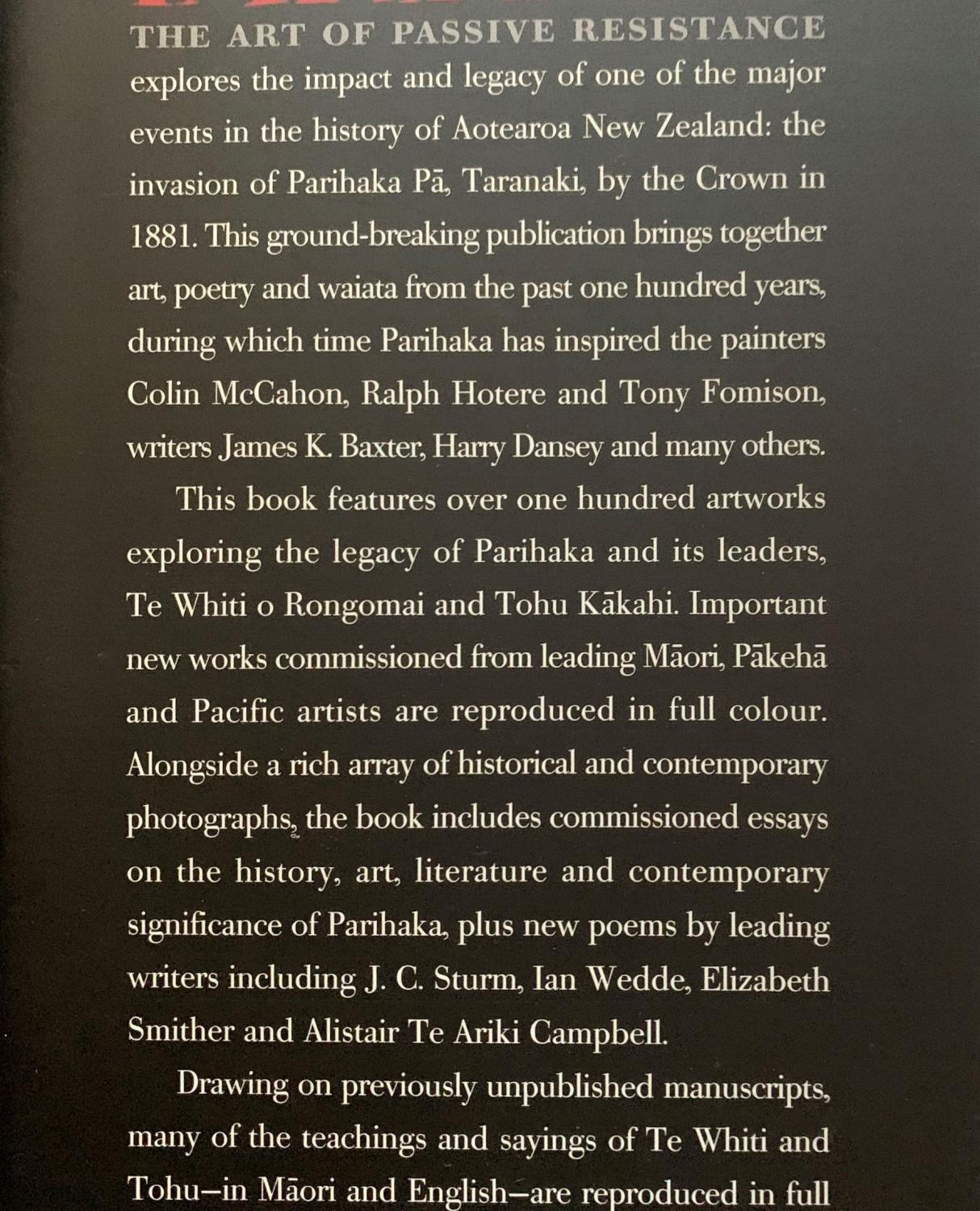The image showcases a dark-colored background — possibly from the back cover or inside jacket of a book — with the title "The Art of Passive Resistance" in prominent text. This book explores the impact and legacy of one of the major historical events in Aotearoa, New Zealand: the invasion of Parihaka Pā, Taranaki by the Crown in 1881. The groundbreaking publication gathers art, poetry, and waiata spanning the past 100 years, during which Parihaka has continuously inspired artists like Colin McCahon, Ralph Hotere, and Tony Fomison, as well as writers such as James K. Baxter, Harry Dansey, and many others. Featuring over 100 artworks, the book delves into the legacy of Parihaka and its leaders, Te Whiti o Rongomai and Tohu Kākahi. It includes important new works commissioned from leading Māori, Pākehā, and Pacific artists, presented in full color alongside a rich array of historical and contemporary photographs. Additionally, the publication contains commissioned essays on the history, art, literature, and contemporary significance of Parihaka, accompanied by new poems from renowned writers J.C. Sturm, Ian Wedde, Elizabeth Smither, and Alistair Te Ariki Campbell. Drawing on previously unpublished manuscripts, many teachings and sayings of Te Whiti and Tohu are reproduced in both Māori and English.